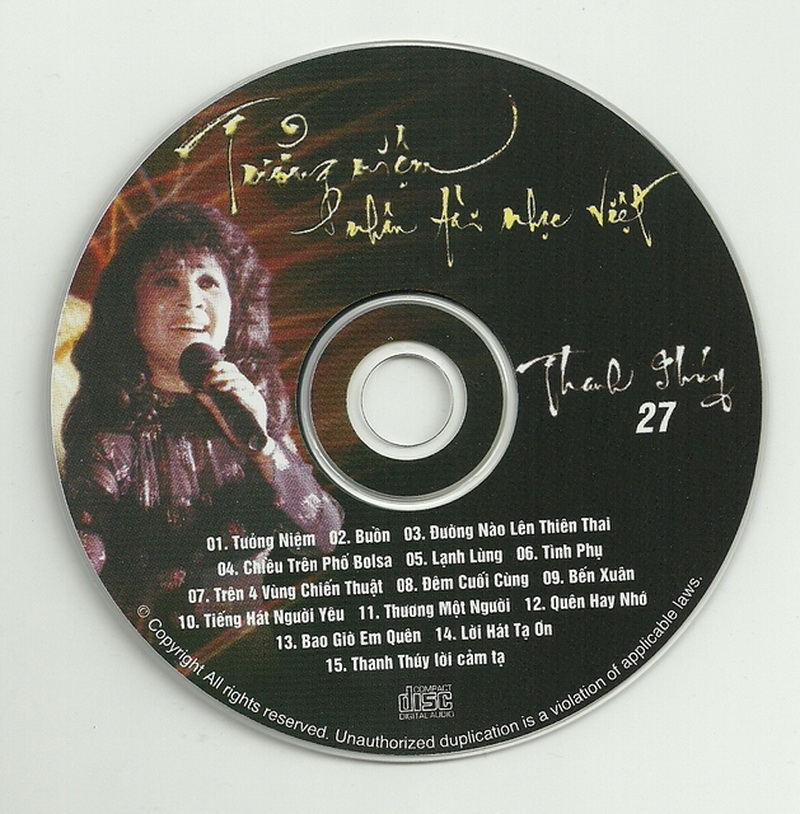This image features a compact disc set against an off-white background, with the CD prominently centered. The disc itself has a primarily black label. On the left side of the label, there's a detailed illustration of a woman with long, bushy, dark hair styled in an 80s fashion. She is captured mid-performance, holding a microphone close to her mouth and wearing a long-sleeved black top. The background behind her transitions into vibrant reds and yellows.

The top center of the CD features hard-to-read handwritten text in yellow, likely indicating a title or the artist's name, suggesting Vietnamese origins given the spelling. To the right of the central image, more white text can be seen, including the number "27" beneath it. Below the central hole, there's a tracklist featuring 15 songs with titles such as "1. Tuong Niem, 2. Buon, 3. Duong Nau Len Thien Thai, 4. Kleu Tren Fo Bol Sa," all written in white. The bottom of the CD reads "compact disc, digital audio," and along the lower rim, the text, "copyright, all rights reserved. Unauthorized duplication is a violation of applicable laws," is printed in white.